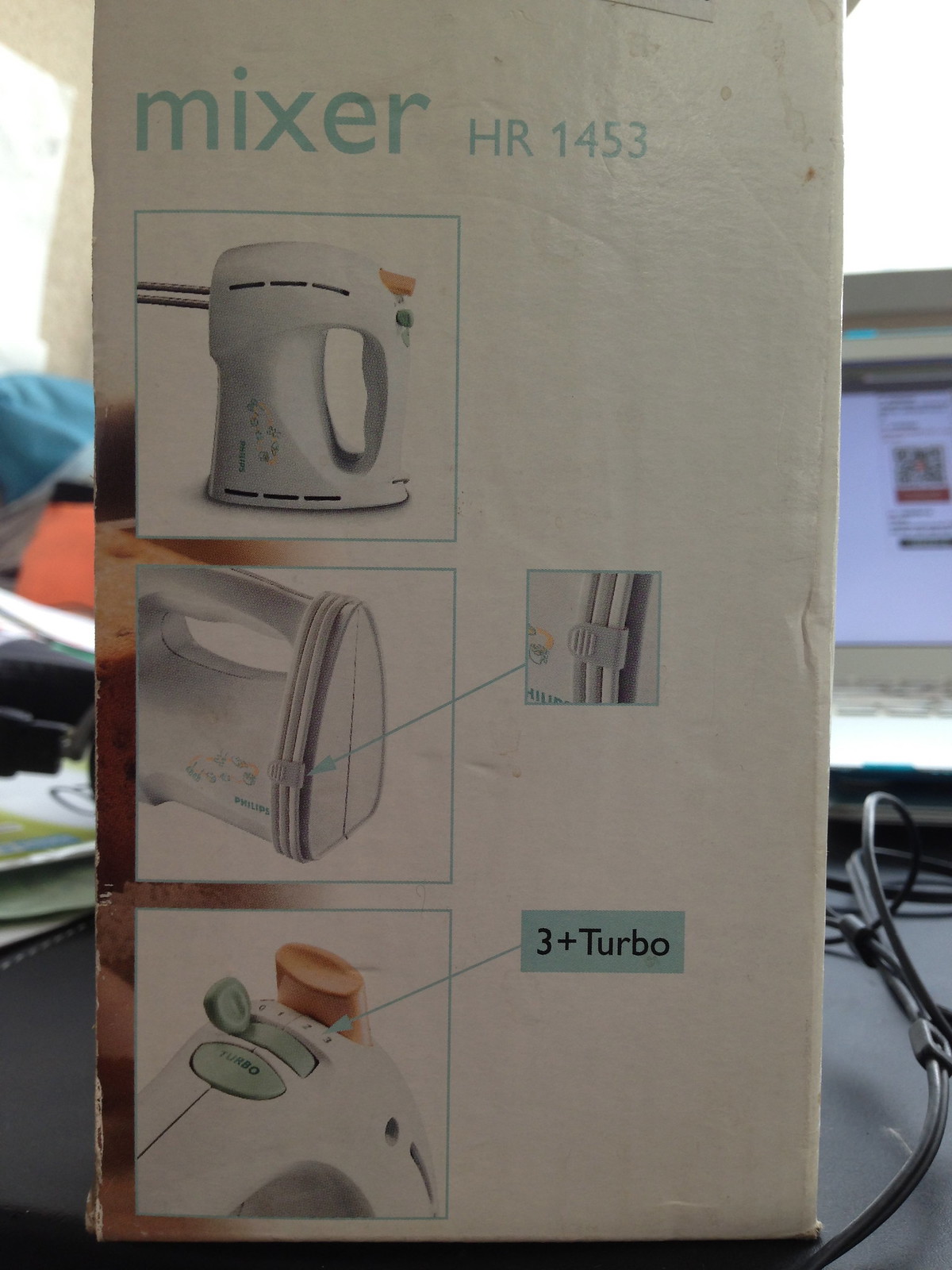This is a close-up picture of a worn-down box for an HR 1453 mixer, with visible stains on the packaging. The box prominently displays "mixer" at the top and features three images of the mixer from different angles along the left side. The mixer itself is white, with a flat bottom and a small, square shape. It has a distinctive hand grip with a hole to place your hand through, and multiple buttons on top, including an orange button and a couple in blue-green hues. One of the images highlights the "3 plus turbo" speed feature. The mixer has a convenient clip for wrapping its power cord. The box is set on a black surface, and the background shows a blurred building and sky. Additionally, there is a laptop and various books and papers visible, suggesting the photo was taken in a home setting.